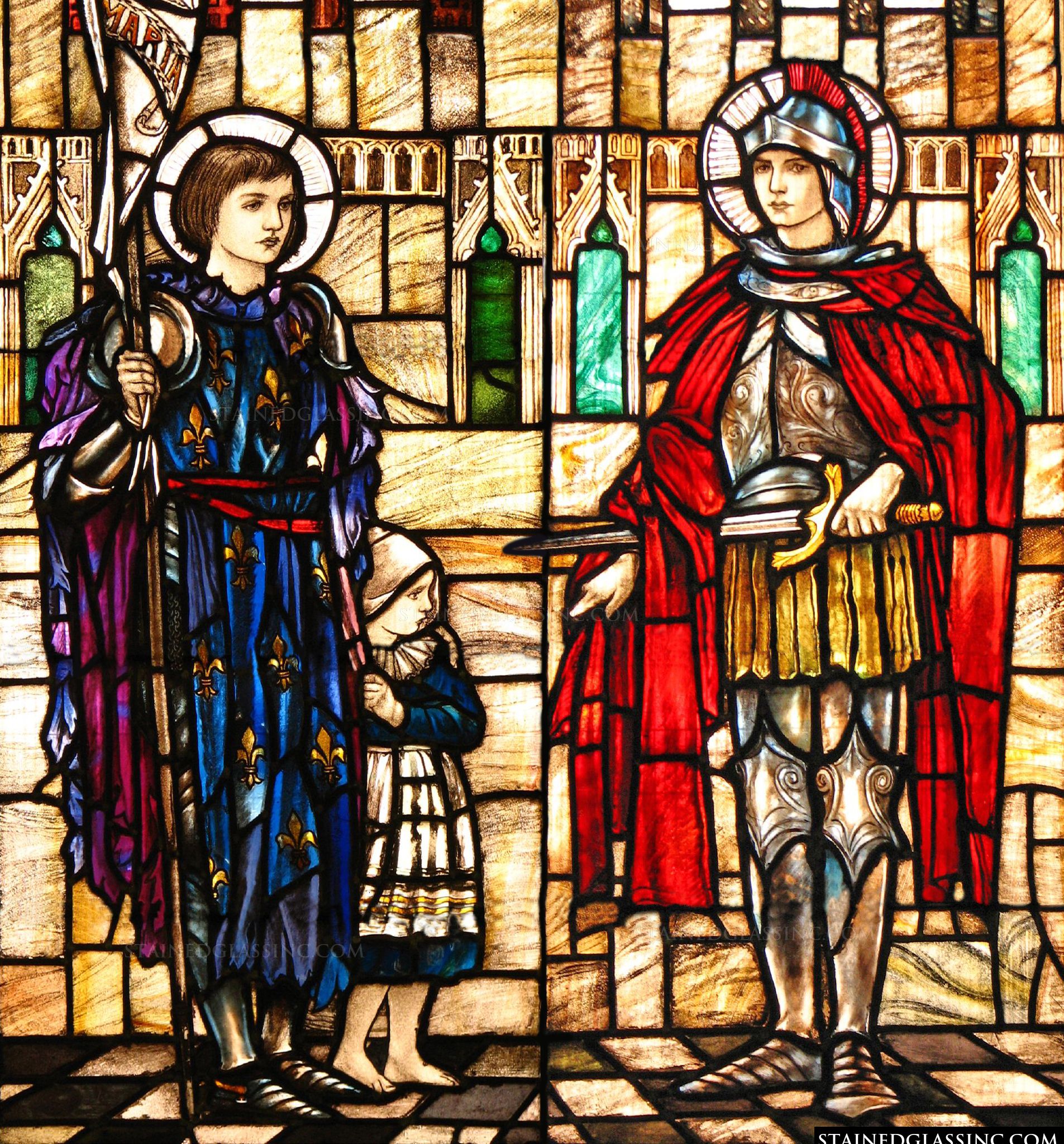This vivid stained glass artwork features a striking scene capturing three figures: a man, a woman, and a child, all illuminated as sunlight filters through the vibrant glass. The man, depicted as a warrior or knight, wears full war armor along with a red robe and holds a sword in his left hand. His blue metallic helmet is adorned with a red plume resembling a Mohican style. Adjacent to him stands a woman in a blue robe with a historical fleur-de-lis pattern; she carries a flagpole with a banner inscribed "Maria." Clinging to the woman’s side is a barefoot young girl, her gaze fixed on the armored man. Both the woman's and the man’s heads are distinctly illuminated, adding a heavenly glow to their forms. The background comprises beautifully colored stained glass, predominantly in shades of beige, lime, and green, enhancing the ethereal atmosphere. In the lower left corner of the image is the inscription "StainedGlassing.com," offering a portal for those interested in exploring more such captivating stained glass imagery.